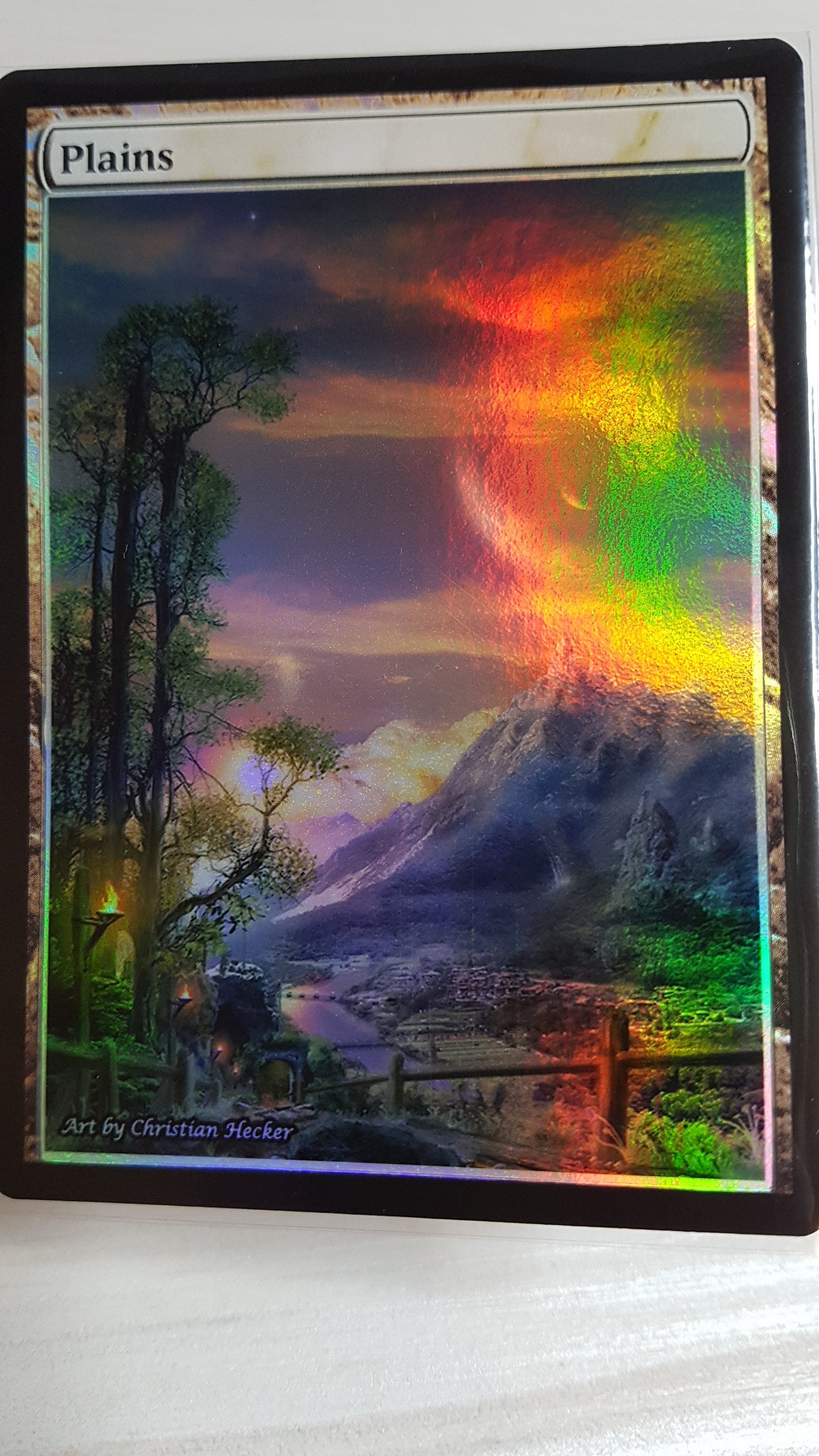This detailed image depicts a full-art Magic: The Gathering card titled "Plains," characterized by its colorful and prismatic elements. The card features a black border and the word "Plains" printed in black at the top left. The central image portrays a vivid landscape, starting from tall trees on the left side, nearly reaching the top where the card's title sits. To the right is a majestic mountain with a light orange and yellowish glow at its peak, complemented by green hues nearby. Below the mountain, nestled in a valley, lies an Asian-inspired village with buildings scattered along a river that meanders through the scene. A wooden fence delineates the foreground, providing a sense of depth as we look out over this picturesque setting. The artwork, attributed to Christian Hecker, is noted in the bottom left corner in a distinctive pseudo-cursive font. The card seemingly lies on a white surface, enhancing the vibrant and magical essence of the depicted landscape.